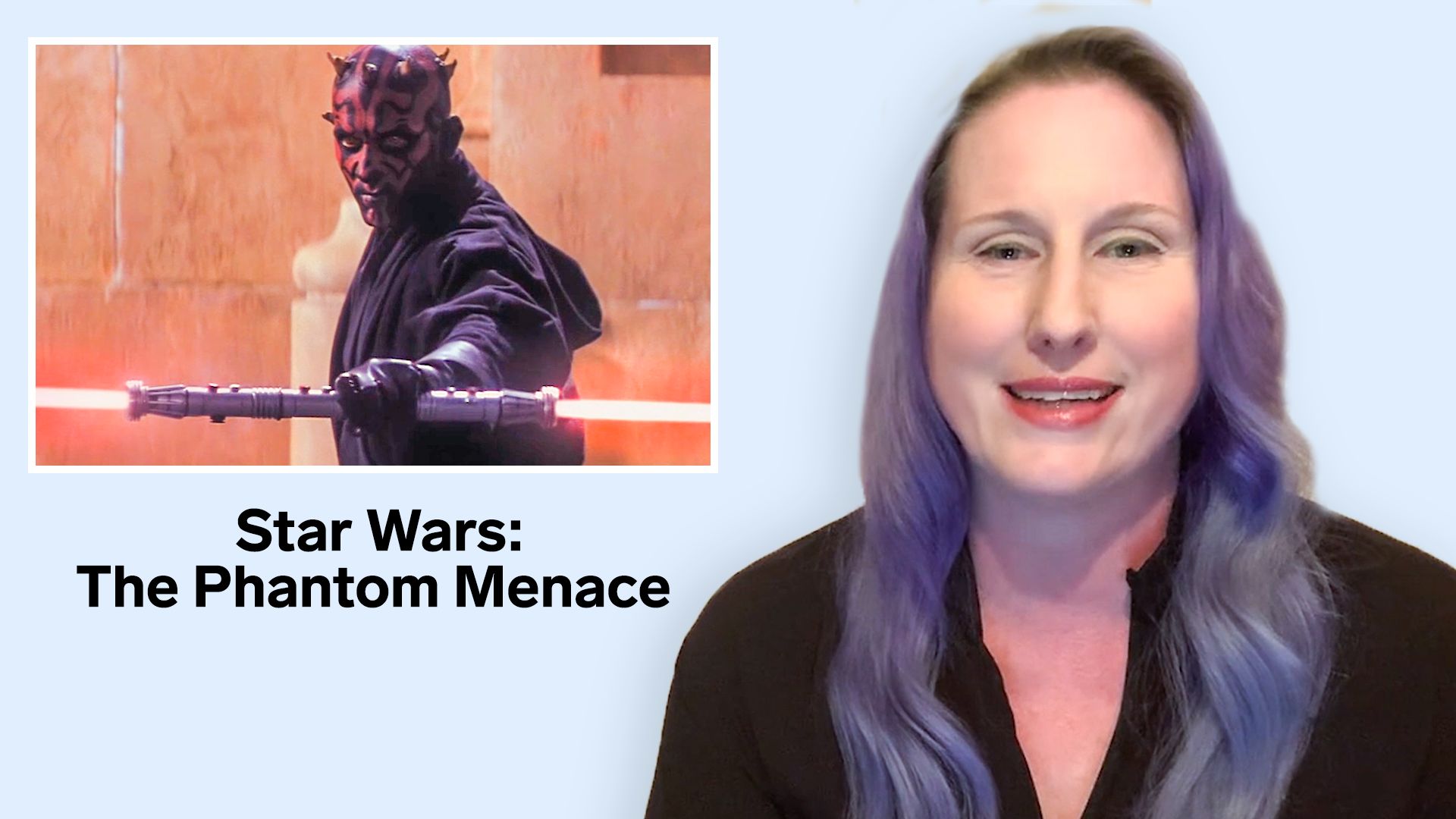This composite image features a horizontally aligned rectangular photograph with a light blue background. On the right side, there's a close-up of a smiling woman, likely in her 40s or 50s, with long hair that is primarily purple, shading to brown at the roots. She has green eyes, light brown eyebrows, and is wearing red lipstick that reveals her teeth. The woman is dressed in a black V-neck top, visible from her chest up, looking directly at the camera.

On the left side of the image, inset in the upper corner, there is a smaller rectangular photograph with a thin white border. This inset picture depicts a Sith warrior from Star Wars, specifically identified from "Star Wars: The Phantom Menace," as noted by the bold black text below it. The Sith character has a menacing appearance, with a red face marked by black lines, small horns, and is dressed in a black hooded robe. He is brandishing a double-bladed red lightsaber, standing against an orange-colored wall that suggests an outdoor setting.